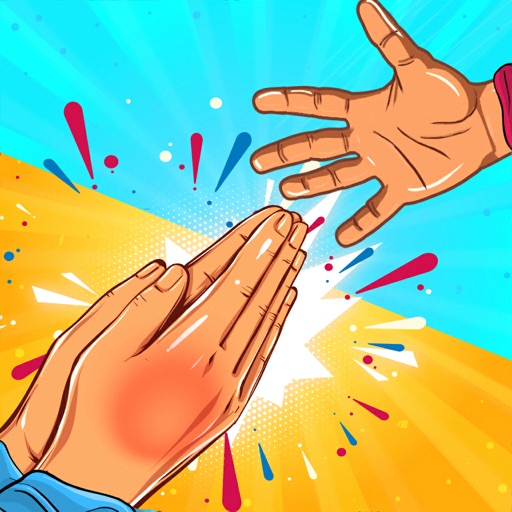In this vibrant cartoon-style illustration, the image prominently features a pair of hands pressed together in a prayer-like gesture, positioned in the lower left corner and extending midway to the upper right. These hands belong to a person wearing blue sleeves, and the right side of the hands appears noticeably red, as if recently slapped. Emanating from the center where the hands meet, dynamic white lines and colorful blue and red exclamation marks punctuate the scene, adding a sense of impact. From the upper right corner, another large right hand with fingers spread wide and palm facing front is depicted, seemingly poised to slap the pair of hands below. The background is split diagonally from the upper left to the lower right, with the top portion colored bright blue and accented by darker blue radiating rays, while the bottom half is a yellowish-gold with orange rays extending downwards, creating a striking dual-colored backdrop.